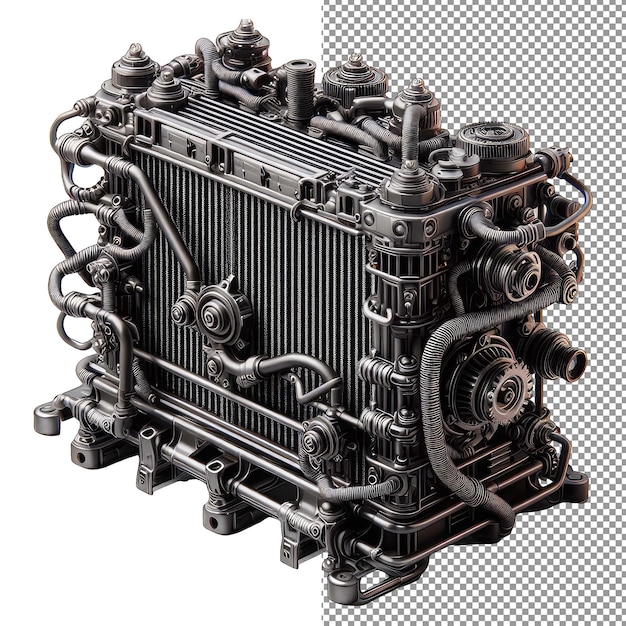This image showcases a pristine, box-shaped piece of machinery, likely an engine or radiator, crafted from matte black metal. The machine, which appears brand new and unused, is adorned with numerous hoses, nozzles, coils, and gaskets, with many vertical lines prominently displayed on its front panel, possibly part of a radiator system. The background is split: the left half is solid white, while the right half features a gray and white checkered pattern, reminiscent of a chessboard or pixelation. This detailed and complex apparatus is highlighted against the contrasting background, suggesting it may have been digitally rendered or professionally photographed.